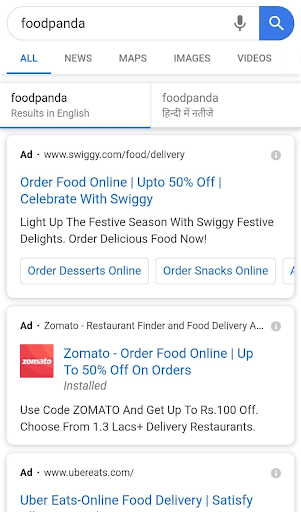This is a detailed caption for an image of a smartphone screenshot depicting a Food Panda web search page:

---

The screenshot displays a smartphone interface showing a web page for Food Panda. At the top, there is a search bar with "Food Panda" entered, complemented by a microphone icon on the left and a search icon on the right. Beneath the search bar, there are tabs labeled from left to right: "All," "News," "Maps," "Images," "Videos." 

Following these tabs, the page features two boxed sections with text: "Food Panda results in English," which is currently active, and a second option labeled "Food Panda" in an unfamiliar language.

Below these boxes, the first advertisement appears for Swiggy.com. The ad text is sky blue and reads:
"Order food online - up to 50% off. Celebrate with Swiggy! Light up the festive season with Swiggy festive delights. Order delicious food now!" 
Two buttons are at the end of this ad: "Order Desserts Online" and "Order Snacks Online."

Following is another ad for Zomato with the header "Zomato - restaurant finder and food delivery," partially cut off. The ad includes the Zomato icon and more blue text:
"Zomato - Order food online. Up to 50% off on orders. Installed. Use code CAPPED OUT ZOMATO to get up to ₹100 off. Choose from 1.3 lakh+ delivery restaurants."

Near the bottom, another ad is partially visible. It specifies that it is for "UberEats.com" with the header in blue text, "UberEats Online Food Delivery," but the rest of the ad content is cut off and only the word "Satisfy" is discernible.

---

This caption describes the contents of the image in a comprehensive and structured manner, covering all the key elements present in the screenshot.